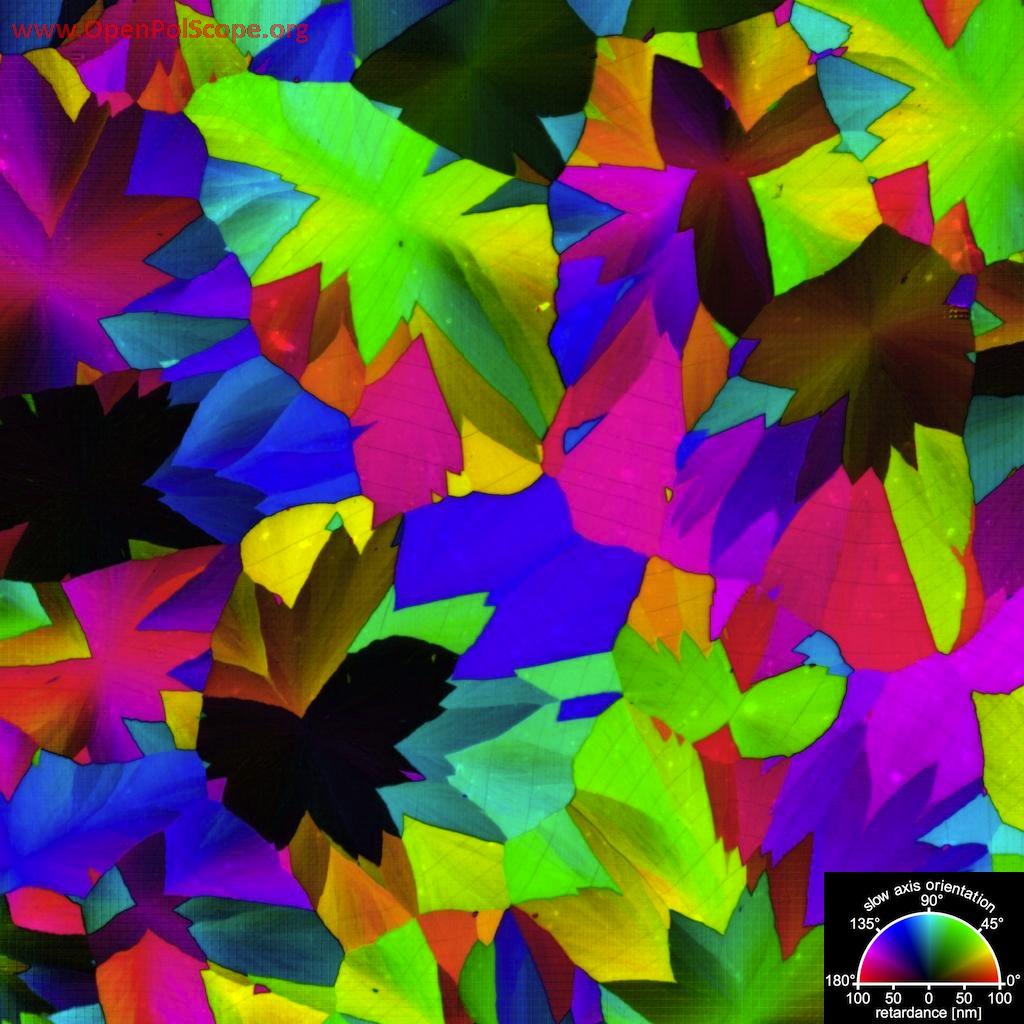The image features a vibrant, tropical-like arrangement reminiscent of patterns often seen on Hawaiian shirts. The design is composed of basic outlines that resemble 3D-generated leaves viewed from above, filled with a plethora of colors including green, purple, blue, yellow, pink, black, and an orangish-brown. In the lower right corner, there is a color control legend, akin to tools used in digital image editing software, allowing adjustment of color values across different degrees for hues such as green and blue. Additionally, a meter at the bottom of the image labels the 'slow axis orientation' and displays a full rainbow of colors ranging from 0 to 180 degrees, alongside a measurement scale for 'retardance' in nanometers (NM). At the top of the image, there is a reference to OpenPolScope.org, suggesting a connection to polarized light microscopy, although the specific purpose of the imagery remains somewhat ambiguous. The varied sizes of the leaf-like shapes add a dynamic feel to the intricate, colorful composition.